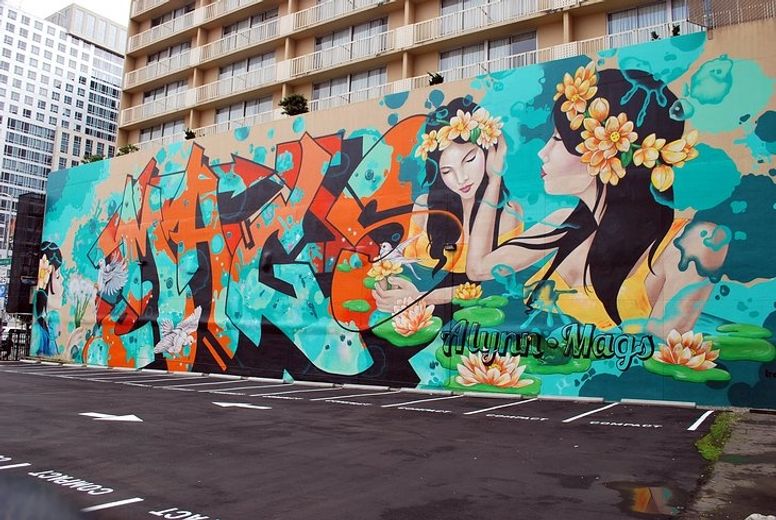The image depicts a vibrant mural on a large wall in a downtown cityscape, likely part of an apartment building or a hotel, given the visible balconies and sliding glass doors above. This six-story-high mural graces an empty black parking lot marked with white lines, designating compact spaces, with approximately 15 spots. Adjacent to the parking lot, there is a tall office building with numerous windows.

Dominating the mural are several women with dark hair, adorned with yellow floral garlands. They appear to have a tropical or South Seas origin, perhaps Hawaiian, accentuated by aqua and blue hues suggesting water and sea themes. Surrounding the women are water lilies in green and orange. On the right side, the name "Alan Maggs" is prominently displayed, while on the left, partially obscured lettering, possibly "Maggs," accompanies an image of a girl blowing dandelions, interspersed with birds. This complex and detailed mural combines professional artistry with graffiti-style elements, making it a striking piece of urban art.